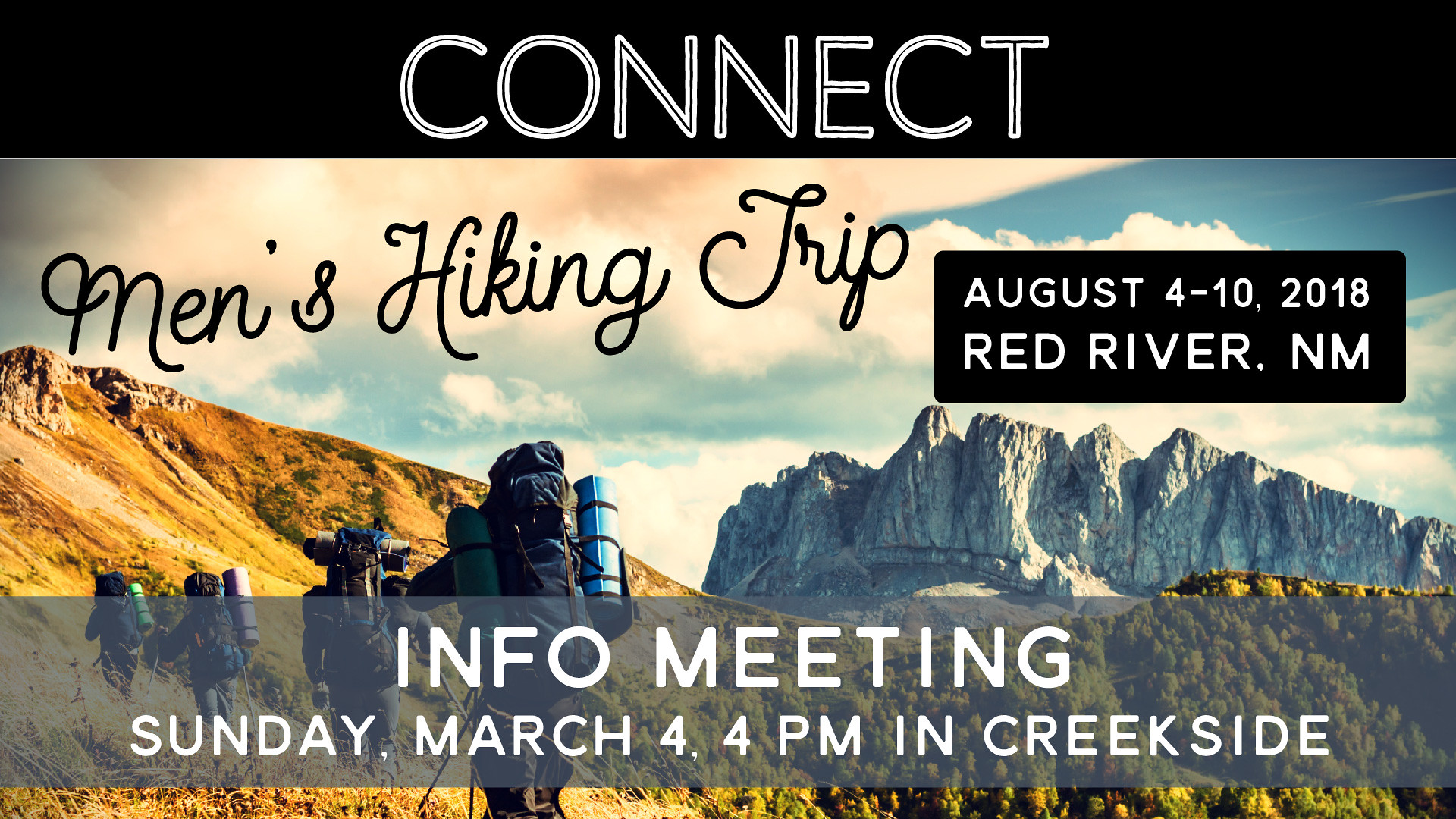The image features a digital poster advertising a men's hiking trip. At the very top, there's a thick black horizontal bar with "Power Connect" written in large white capital letters. Below this bar, a vivid, full-color background photo shows four hikers ascending a lush, green mountain with towering white cliffs to the right. The hikers are equipped with large backpacks and sleeping pads. Superimposed on this scenic background, to the left in black cursive is the text "Men's Hiking Trip," and to the right, inside a black rectangle with white text, the dates "August 4-10, 2018 Red River, NM." At the bottom of the poster, a translucent light blue or gray horizontal bar displays in white text: "Info meeting Sunday, March 4, 4 p.m. in Creekside."